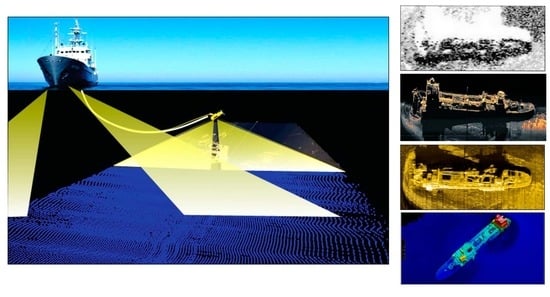The image is a blue-themed graphic art illustration prominently featuring a large rectangular section on the left and a vertical strip of four smaller images on the right. The main section showcases a steel-gray blue ocean liner with a white cabin atop, complete with visible radar machinery and a windsock, positioned against a background that transitions from sky blue at the top to white near the horizon. Below the vessel, a royal blue area resembling a dock extends over a much darker blue, likely representing the ocean. This royal blue area includes gold triangles connected by lines, symbolizing anchors or hitch posts.

The four smaller images on the right consist of:
1. A black and white depiction of water splashing against rocks.
2. An aerial view of a battleship.
3. Another aerial view of a battleship in a yellow-toned setting.
4. A neon blue ship on dark blue water.

These images may represent shipwrecks or various ship-related scenes, illustrating maritime themes.